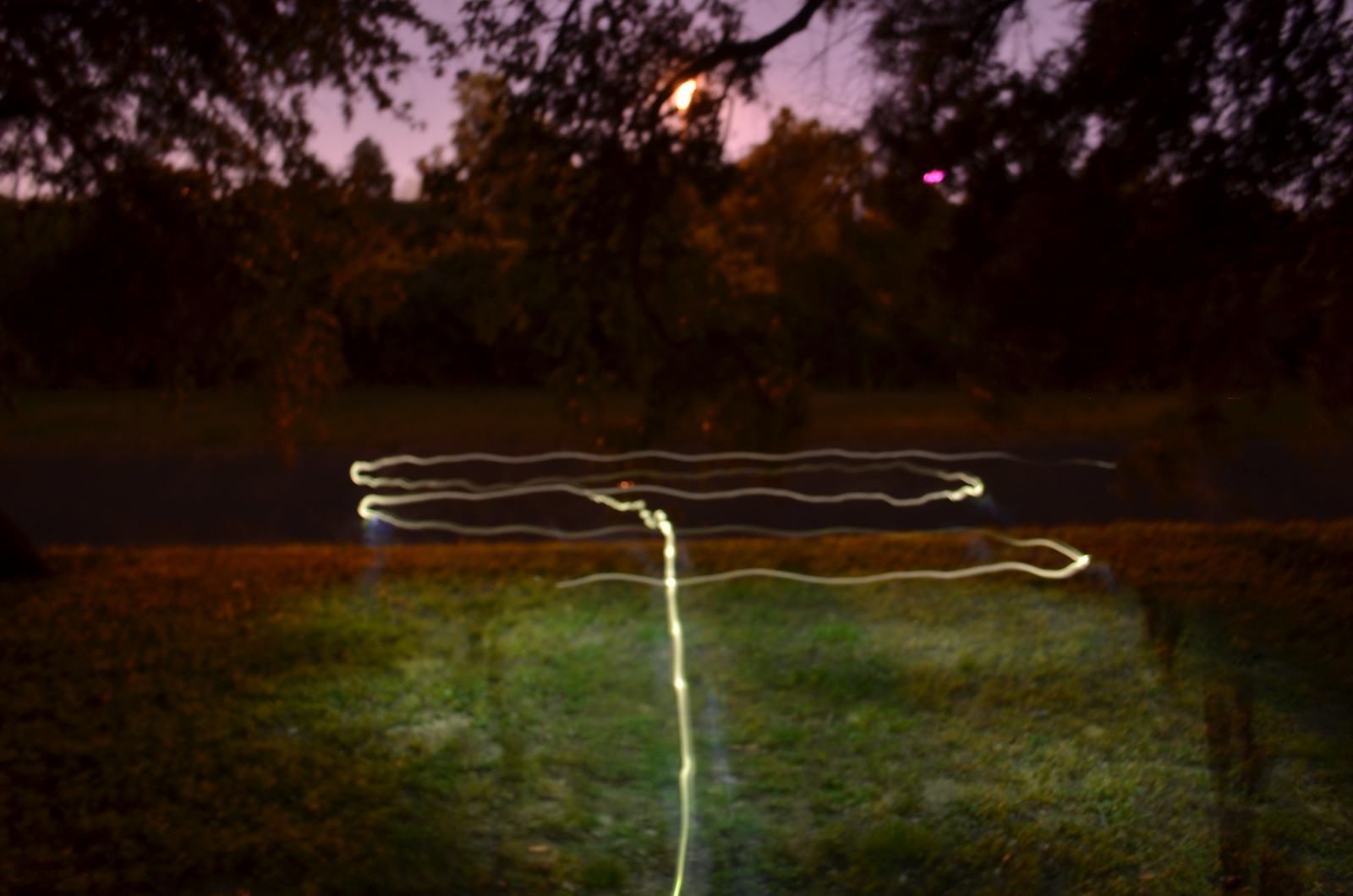The photograph captures a serene outdoor scene during sunset, where the sky is painted in a beautiful, very light lavender or pale lilac hue. The sun is setting behind a line of trees in the center of the image, creating a subtle glow. The foreground features lush, green grass and possibly a body of water, adding to the tranquil ambiance. There's a paved road cutting through the middle ground, bordered by greenery and trees with vibrant green leaves.

A striking feature of the image is the mysterious light phenomenon near the bottom center. It appears as a thin, white line resembling an electrical current or a glow from a laser light, creating a mesmerizing effect as it spirals and squiggles through the air. This light forms two or three circular loops, similar to a cowboy’s lasso, and illuminates the surrounding grass. This intricate pattern, possibly captured using time-lapse photography, gives the scene an ethereal and almost otherworldly quality, making it both captivating and enigmatic.